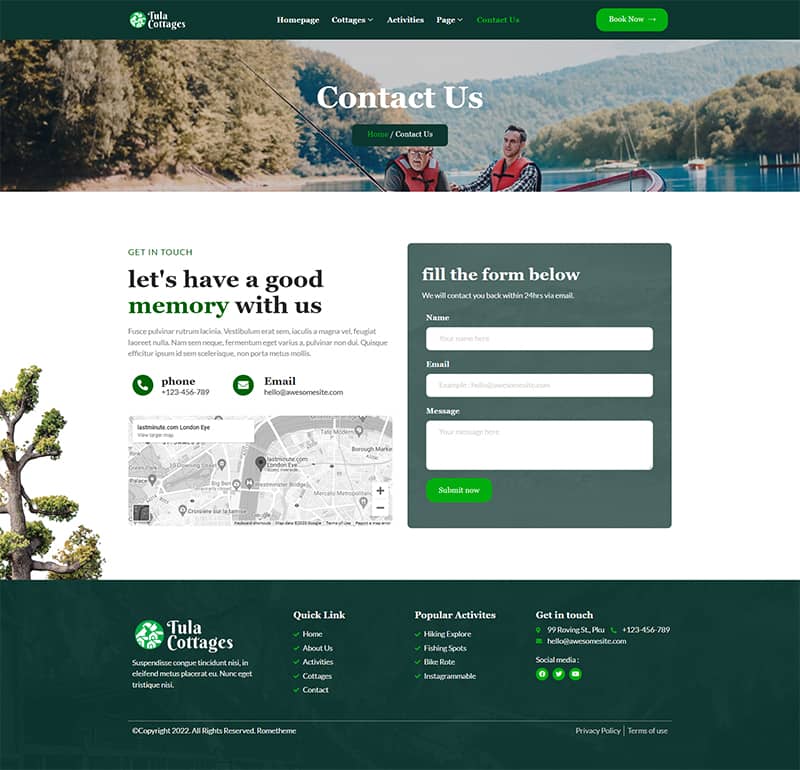**Caption:**

This image is a detailed screenshot of the Tula Cottages website. The topmost section features a dark green banner adorned with the Tula Cottages logo in white text on the top left, accompanied by a circle containing small cottage icons. The navigation menu includes tabs labeled "Homepage," "Cottages," "Activity Page," "Contact Us," and a "Book Now" button in light green with white text. The "Contact Us" tab is highlighted in dark green, indicating it is currently selected. 

Just below the banner, a partially visible photograph depicts an older man and a younger man fishing in a boat on a river, surrounded by water and trees. The image cuts off their lower bodies and most of the boat. Underneath this picture, there’s a white form headed by the text "Get in touch, let's have a good memory with us," with the word "memory" highlighted in green. A brief, somewhat unreadable paragraph of gray text follows.

Directly beneath, you’ll find icons for a phone number and an email address, along with a gray-toned Google Maps thumbnail showing a pinned location. To the right, a dark green box with white text invites visitors to "Fill the format below, we will contact you back within 24 hours via email." The form includes fields for the user’s name, email, and message, followed by a light green "Submit Now" button.

The bottom of the screenshot displays a large green rectangle with quick link navigation options for ease of browsing the website. To the left of the "Get in touch" section, a part of the image shows a section of a tree, adding a natural touch to the page’s design.